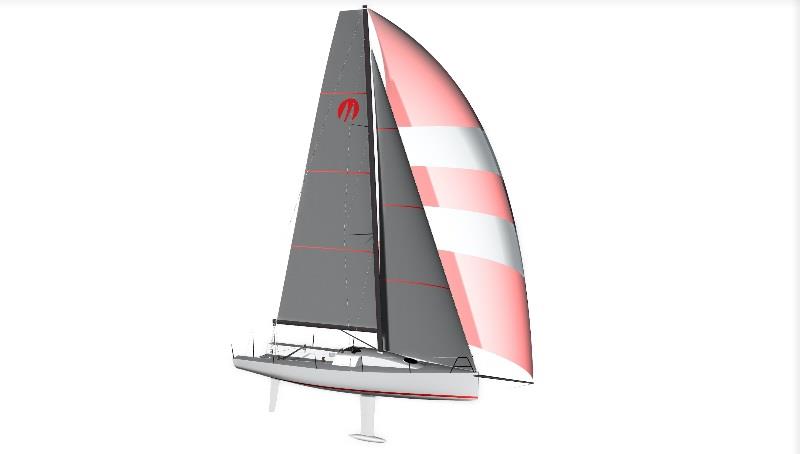The image is a 3D graphic representation of a keelboat, set against a completely white background. The boat itself has a light grey hull with a distinct red line running along the bottom, and the deck is a darker grey. A tall mast rises from the deck, supporting three sails. The foremost sail is dark grey with three small horizontal red lines and a logo resembling a red 'M' within a circle at the top. Behind it is another grey sail, similar in design but slightly larger and more triangular, also adorned with horizontal red stripes. The third sail, positioned to the right, is pink with two thick horizontal white stripes. The sailboat also features a propeller underneath and a glide fin extending from the bow, further enhancing its detailed design.